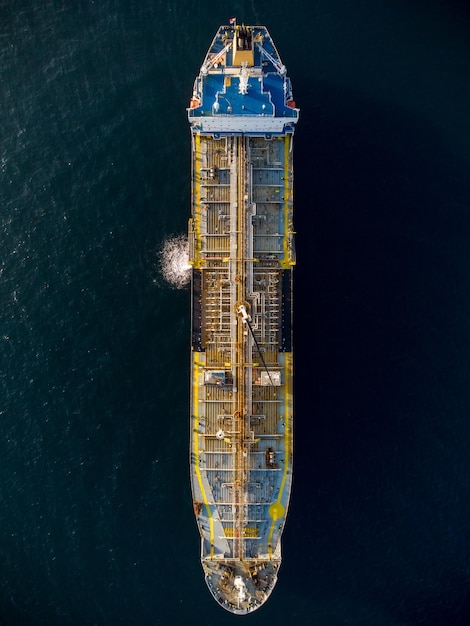This overhead aerial photograph captures a large cargo ship navigating through dark blue, almost black waters, with sunlight slightly illuminating the left side of the scene. The ship spans the entire vertical space of the image, emphasizing its impressive size, as the people on board appear as mere dots. The ship features a distinct blue deck at the nose, contrasted by a similar blue area at the rear. The deck is predominantly laden with what looks like wooden materials, presenting a palette of beige, brown, yellow, and blue. A striking feature is the white crane situated centrally on the vessel, extending outward with its black crane arm pointing towards the bottom right. Additionally, water is seen being discharged from the ship's left side, creating a foamy white disturbance as it meets the ocean surface below.